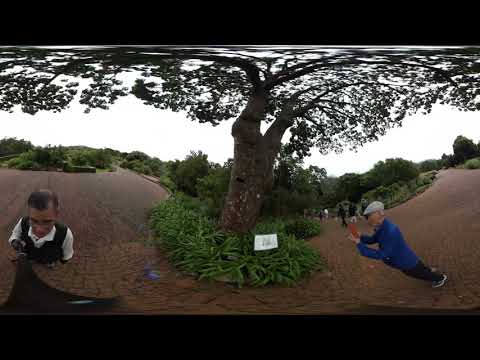In the image, we see a panoramic view centered around a large tree whose leaves extend towards the edges of the image, creating an illusion as if they are bending down against an invisible glass ceiling. The tree is surrounded by various shrubs and bushes, with a small white sign among the vegetation at its base. The surface around the tree is a brownish-dark color, resembling a brick or paved walkway.

On the left side of the image, a man is holding a selfie stick in his right hand, which appears on the left to the viewer. He has black hair around a balding top and wears glasses. His attire includes a black vest over a white button-up shirt. He is looking down at the camera. Behind him, the ground is a brown brick-like walkway, with some shrubbery and square bushes visible.

To the right of the tree, another man is in the process of taking a picture. He is dressed in black pants, a blue shirt, and a small white beanie. Due to the panoramic effect, the image distorts, making him appear to be leaning at a sharp angle, almost 45 degrees to the ground. The background includes more people walking along a curved path, with additional trees framing the scene, creating a lively and natural environment.